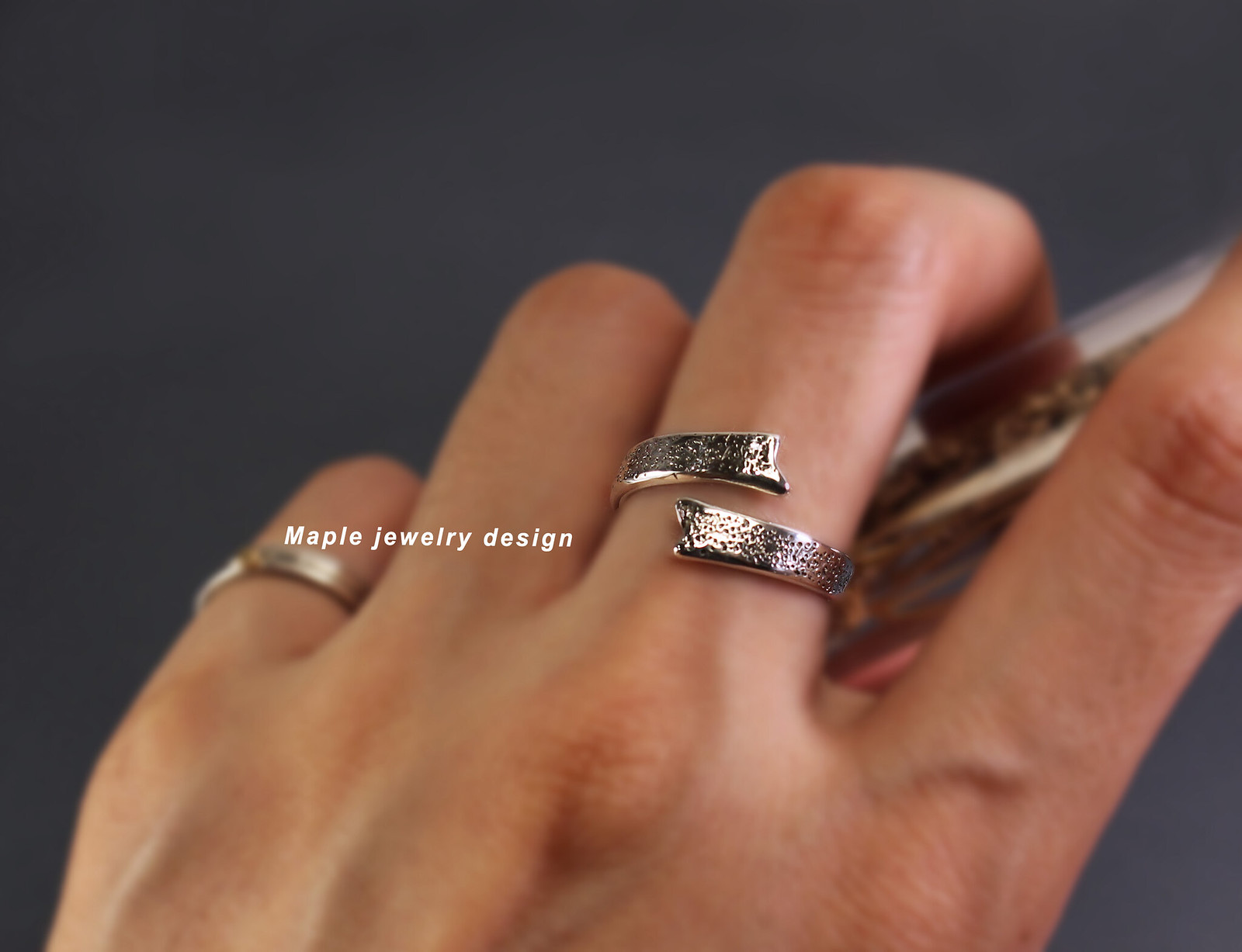The photograph showcases a close-up of a partially visible left hand adorned with rings, set against a featureless, solid dark grey background that gives the hand an impression of floating in a void. The focal point is the rings on the hand, particularly the distinctive ring on the middle finger. This ring exhibits a unique design where the band is intentionally broken, leaving two overlapping segments that do not connect. The ends of this metallic silvery ring, textured with tiny holes, appear as if they have been torn apart. A simpler, traditional gold-colored ring graces the pinky finger. Overlaying the hand is white text reading "Maple Jewelry Design," adding a minimalist accent to the composition.